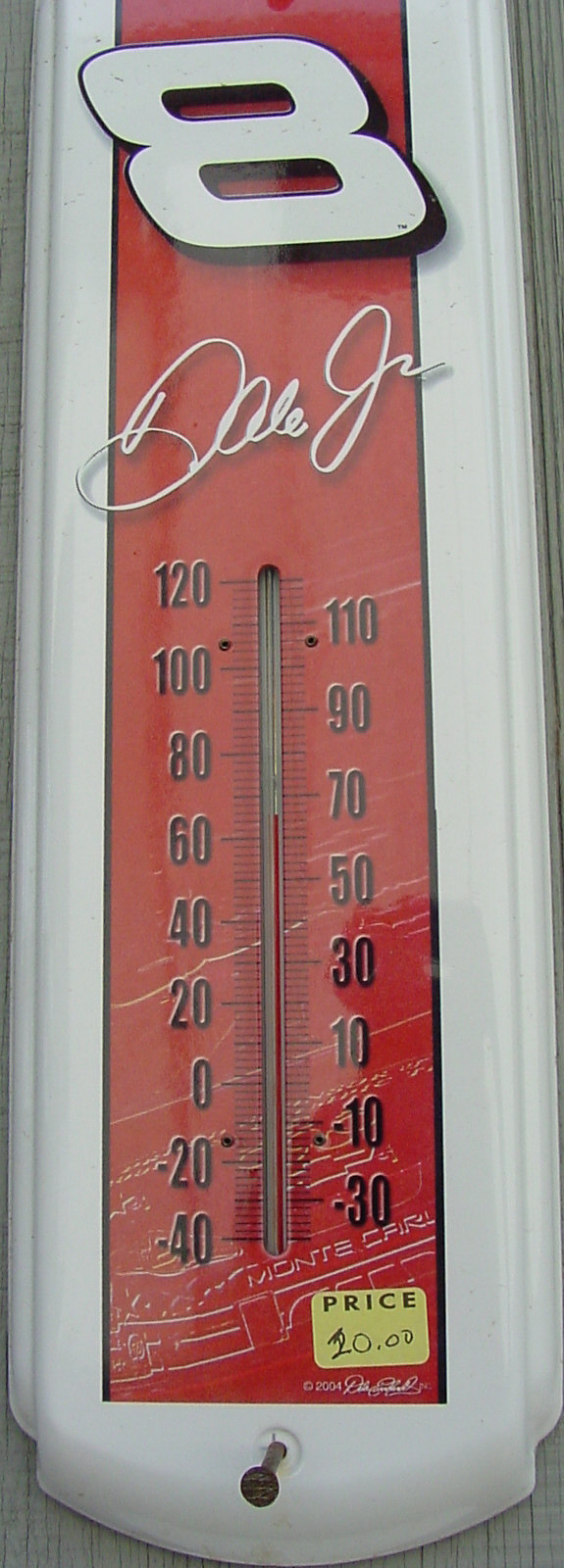This photograph features a vintage or collectible white thermometer mounted on the side of a wall with a nail near its bottom. The frame of the thermometer is white, and it prominently displays a red vertical section along its center. Positioned at the top of this red area is a white number "8," followed by the cursive text "Dale Jr.," which likely refers to NASCAR driver Dale Earnhardt Jr. The thermometer itself, located below this text, has dual temperature scales. On the left side, the scale reads 120, 100, 80, 60, 40, 20, 0, -20, -40, while on the right side it reads 110, 90, 70, 50, 30, 10, -10, -30. The bottom of the red section features a yellow sticker with the word "price" in black text and a handwritten note indicating the price as $20.00. The top portion of the thermometer is cut off in the photograph.